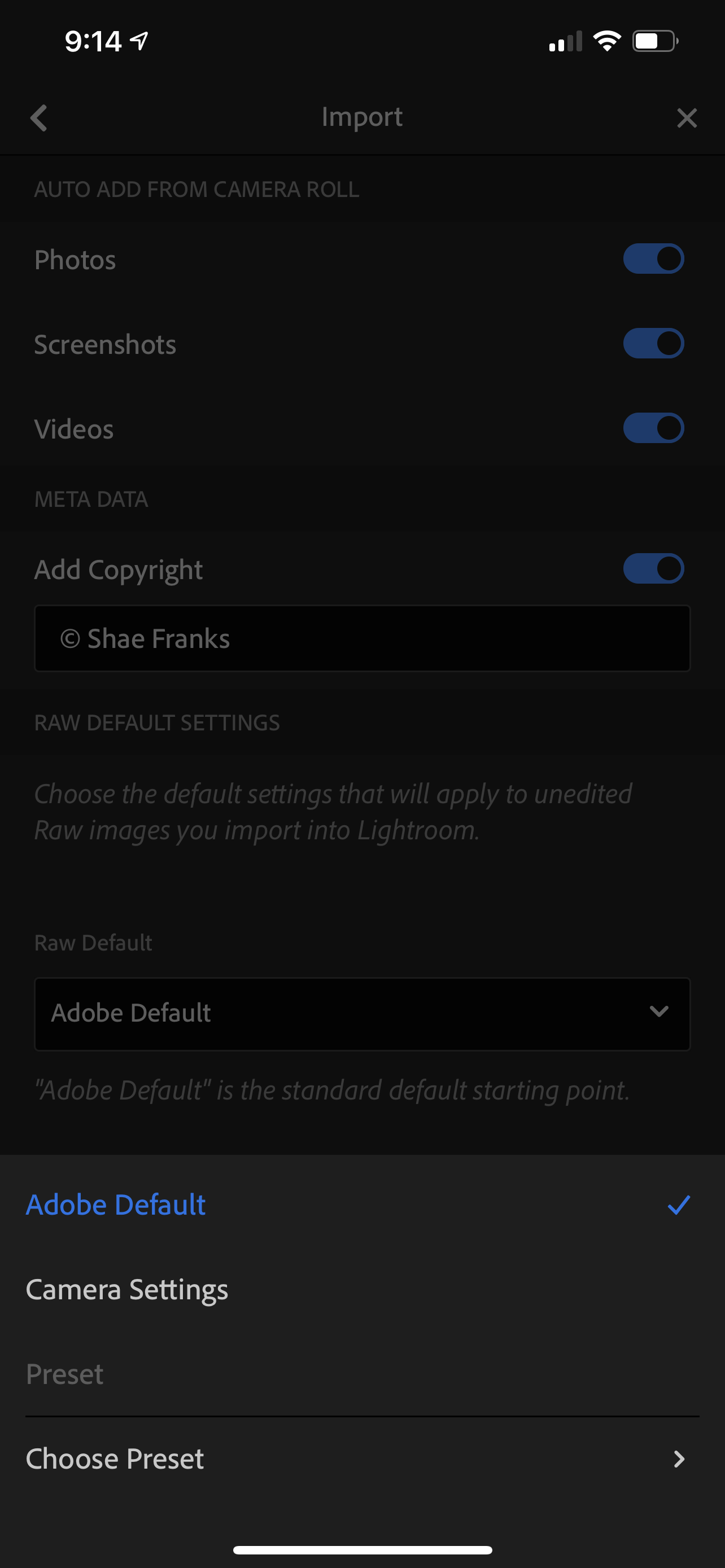The image appears to be a screenshot taken on a smartphone, featuring a predominantly black interface. In the upper left corner, the time reads "9:14" in white text, while the battery icon on the top right shows approximately 75% charge.

Just below, there is a search bar labeled "Import." Below this search bar, several toggles are visible, all switched on, for "Photos," "Screenshots," "Videos," and "Add Copyright." The text "Shea Franks" appears directly beneath the "Add Copyright" toggle, suggesting it might be the name associated with the imported media.

A lighter gray section follows, containing text that is difficult to decipher. Beneath this, a black search bar displays "Adobe Default" in blue, accompanied by a drop-down arrow on the right side. The bottom section of the screen transitions to a gray background, where "Camera Settings" and "Preset" are listed in white text. The words "Choose Preset" are followed by an arrow on the right, indicating a clickable option for further choices.